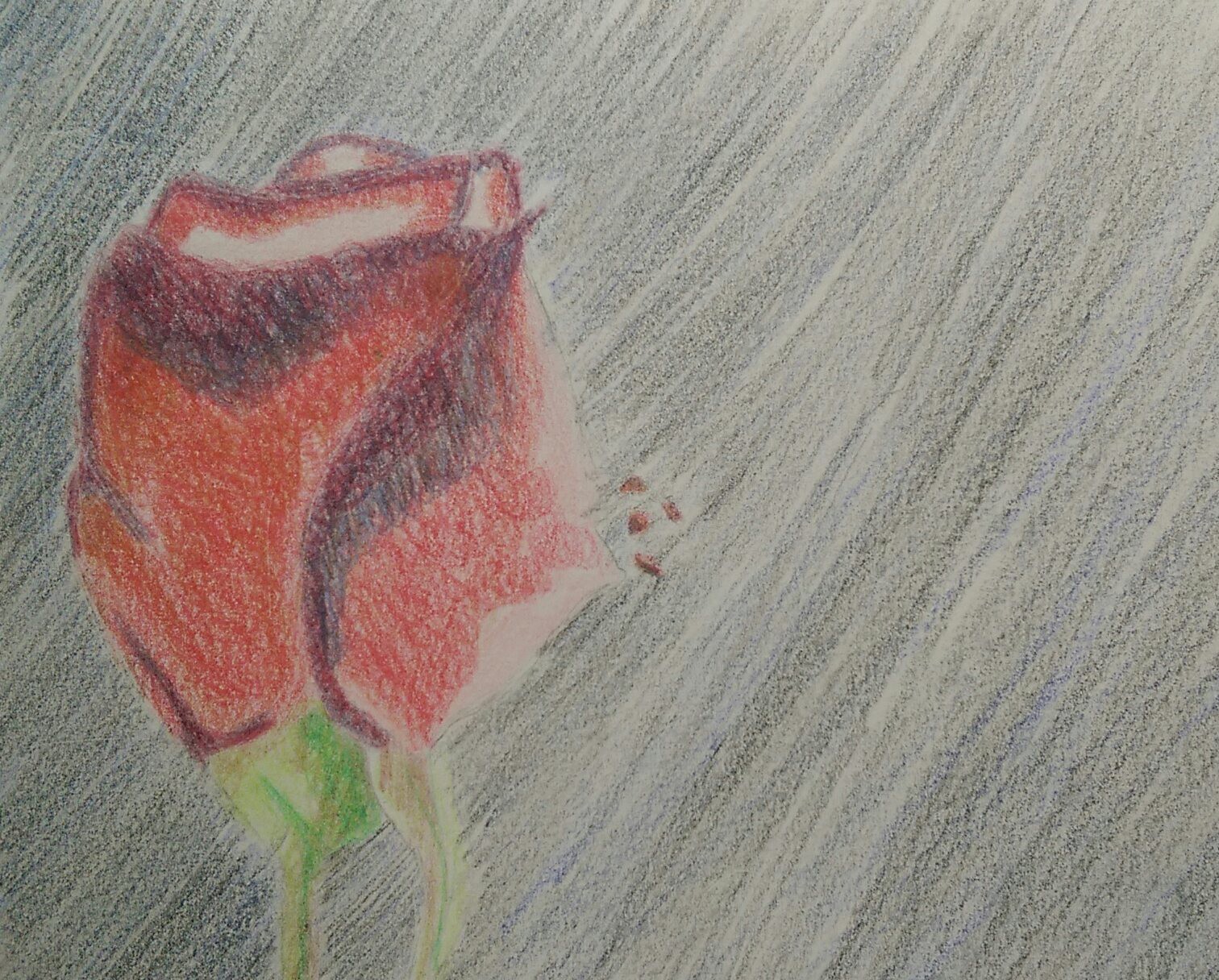This image features a detailed colored pencil drawing of a partially open red rosebud, positioned near the left side of the composition. The rose, not fully open, displays intricate layering of petals with varying shades of red, from lighter pinkish hues to dark maroon edges and white highlights. A light green stem, accented with brighter lime highlights on the right side, supports the rose, accompanied by a subtly visible green leaf extending downwards. Four small red dots are neatly arranged to the right of the rose. The background consists of lightly shaded sketch lines in black, blue, and gray, arranged diagonally and creating an impression of rain. The overall texture of the rose and its surroundings is vividly conveyed through the meticulous pencil strokes, granting the image a lifelike yet artistically abstract quality.